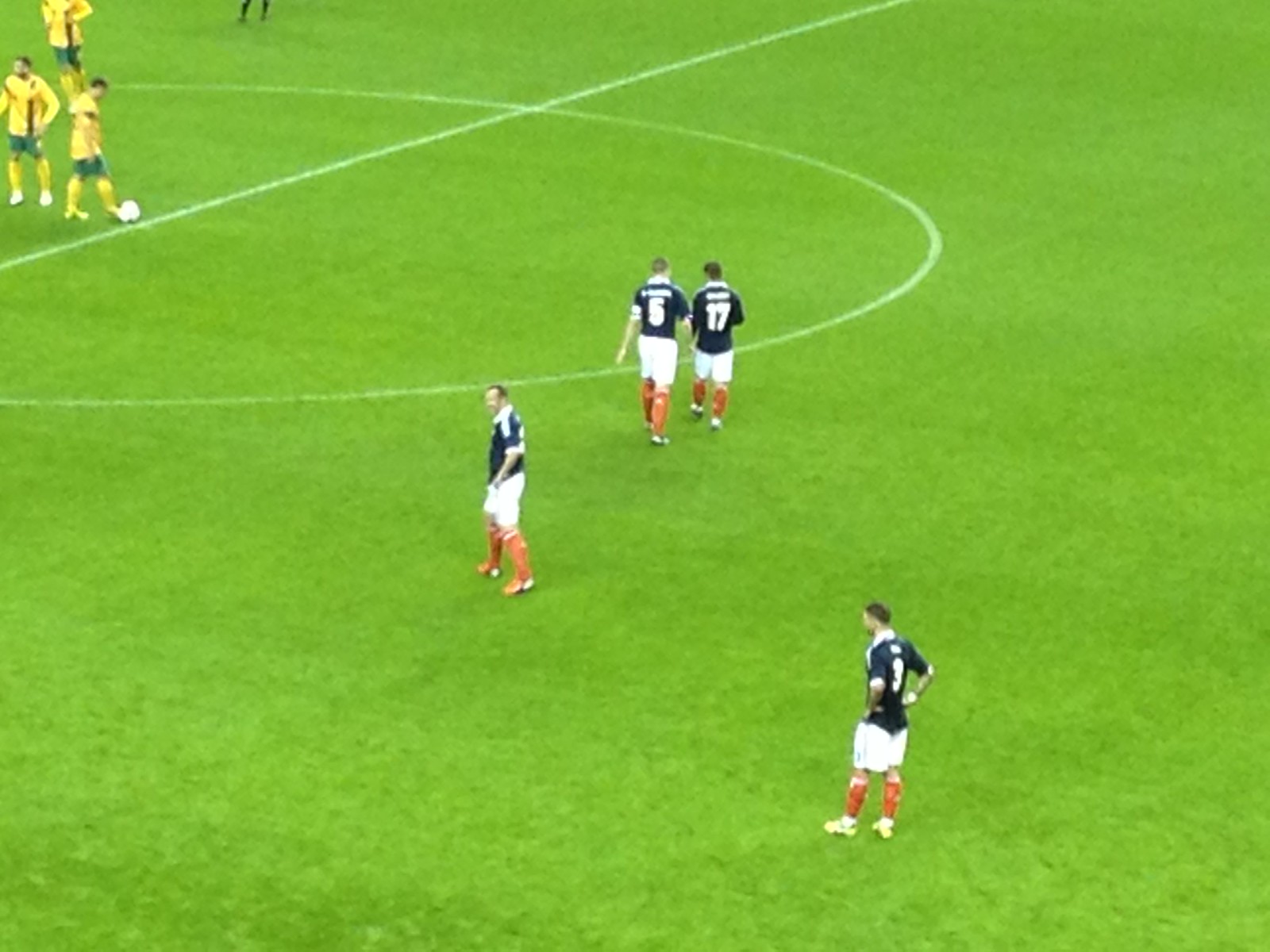The image captures a paused moment in a soccer game on a bright green field with clearly defined white boundary lines, including a large circular midfield marking. In the foreground, four players wearing dark green (possibly black) jerseys with white shorts and orange socks are preparing for the next play. To the left, three players in yellow jerseys, green shorts, and yellow socks are gathered, one of whom has his foot on the ball, seemingly setting it up for a kick. The scene suggests a potential midfield setup or a free-kick situation. The blurred background contains partial images of additional individuals, possibly players or referees, indicated by visible legs in the upper left corner.